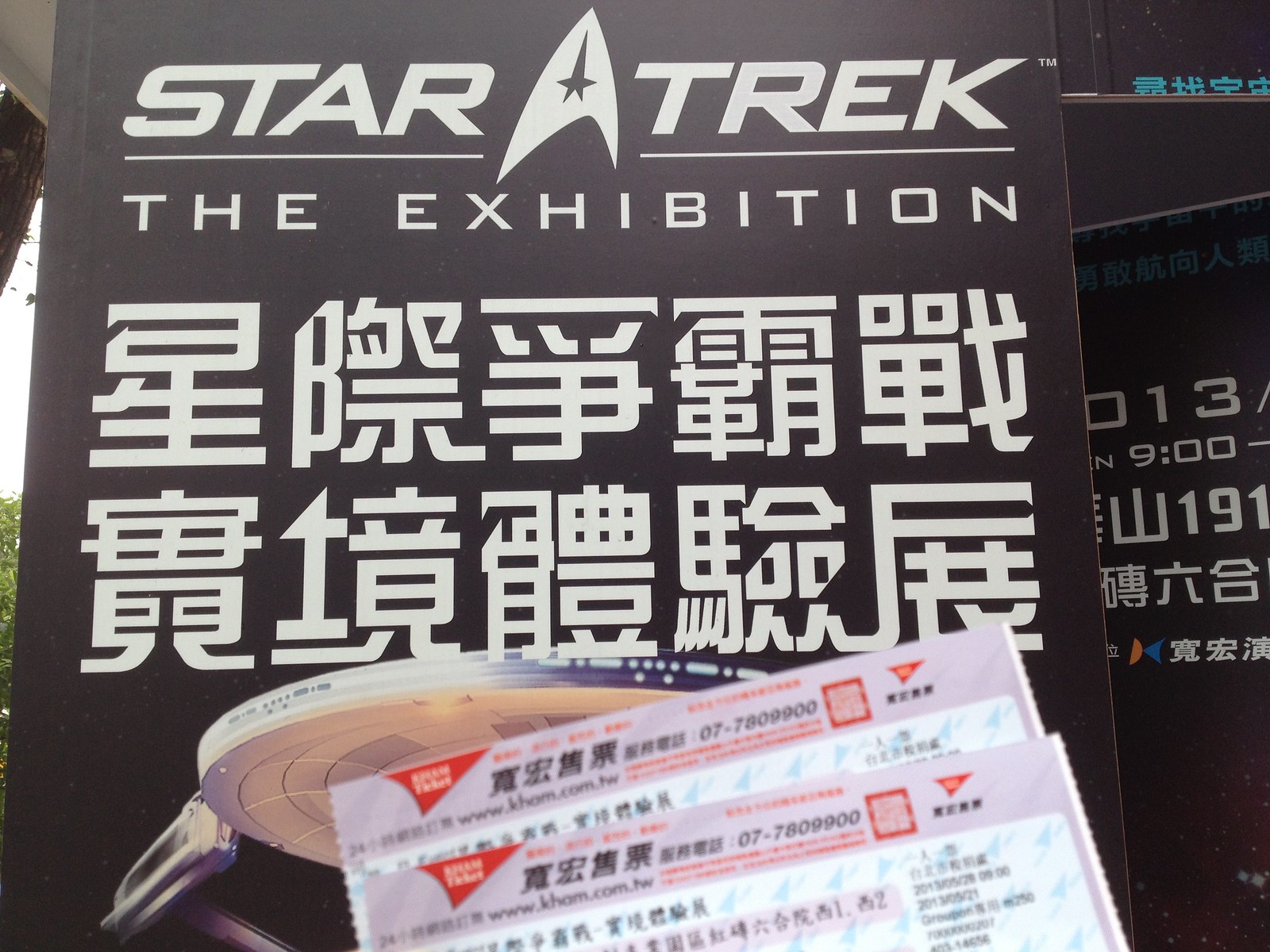The image features a large, black display banner with white text that prominently reads "STAR TREK THE EXHIBITION" in capital letters, showcasing the iconic Star Trek logo, which has an arch-like design. Below the main text, there are two lines of Asian characters, also in white. The display seems to serve as an entrance or promotional sign for a Star Trek exhibition, likely held in a museum. Partially covering the starship graphic on the banner are two tickets, which are pink and white with blue repeating patterns, suggesting they are for this event. The photograph appears to be taken outdoors, evidenced by the visible white sky and some green leaves in the background.